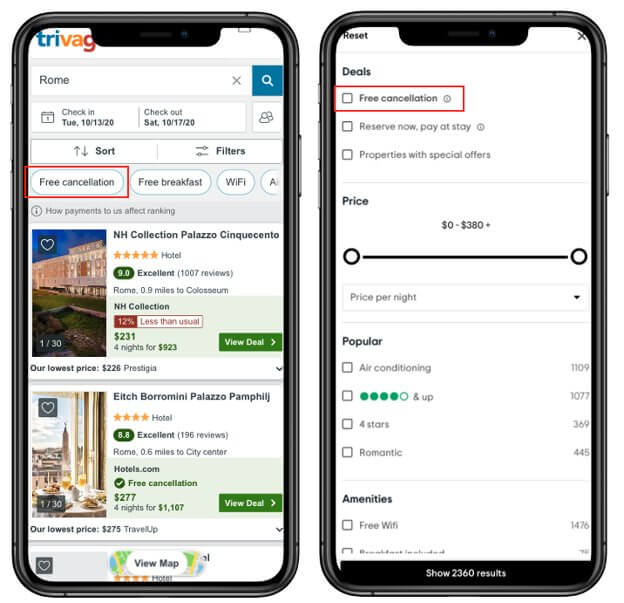Two cell phones are displayed side-by-side in the image. The phone on the left shows a Trivago app screenshot, clearly highlighting the "Free Cancellation" option within a red box. Similarly, the phone on the right features the "Deals" app with the same "Free Cancellation" option, also emphasized with a red box. Both screen displays focus on emphasizing the availability of free cancellation for bookings.